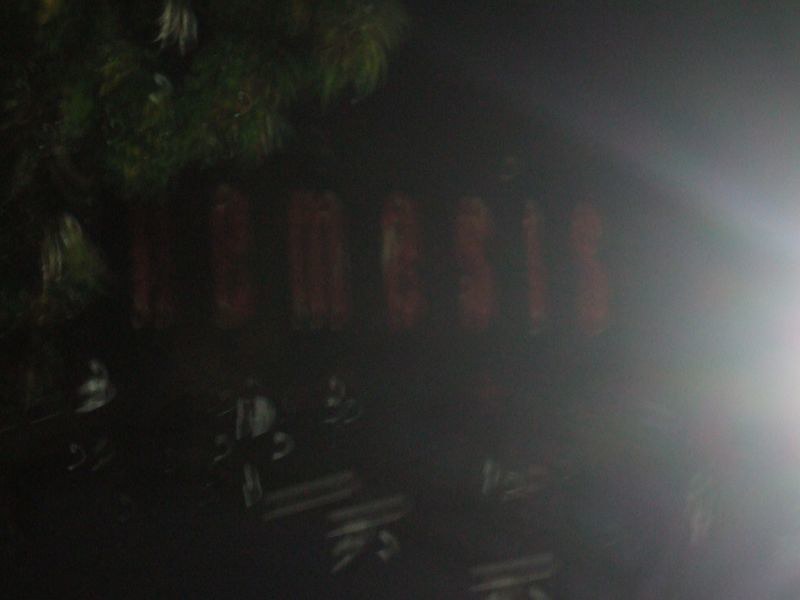In the top left corner of the image, lush green leaves add a touch of natural vibrancy. The background features a mix of vivid red hues, adding depth and contrast. On the right side, a bright white light dominates, creating a striking focal point. The bottom portion of the image is illuminated with a subtle, ambient lighting that adds a soft glow. Surrounding the main elements, various shades of black provide a dramatic framing. The bright white light on the right has a slightly blurry effect, creating intriguing visual marks that carry through from the top left to the middle and bottom of the image.